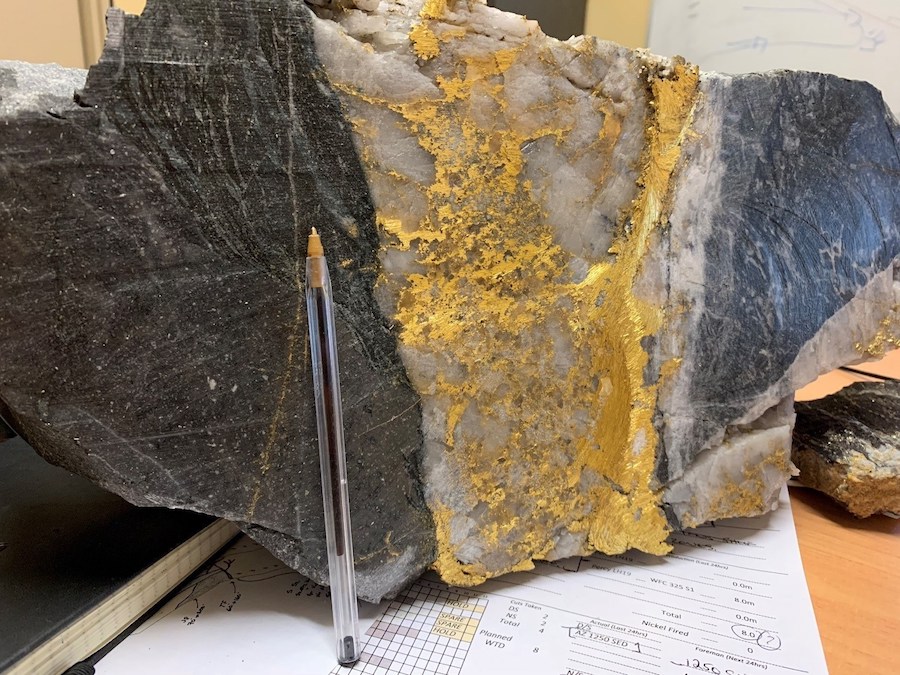The image displays a slab of rock positioned on a piece of paper, accompanied by an ink pen standing tipside up in front of it. The rock features a striking array of gold deposits, with multiple spots, strands, and patches predominantly concentrated in the middle white, marble-like section. The left side of the rock is dark gray, accentuated by a thin gold line, while the right side exhibits a slight crack forming a V-shape at the bottom, also dark gray in color. The setting includes additional items such as a book and other objects positioned to the side, suggesting a contextual background of study or examination.